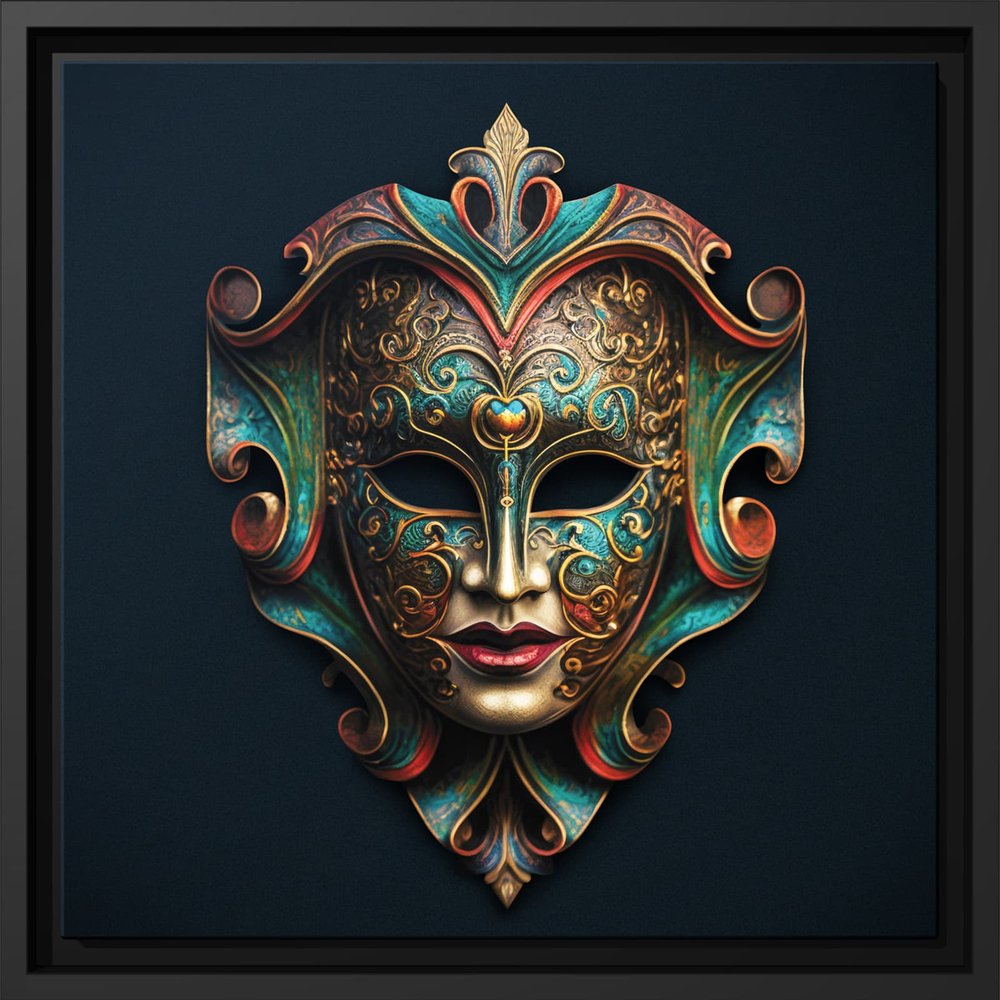The image showcases a highly detailed and vibrant artwork of a metallic mask, framed in black against a dark midnight blue backdrop. The mask resembles the face of a woman, with human-like red lips vividly painted, giving it a lifelike appearance. The mask features hollow eye cutouts and intricate gold filigree swirls across its surface. Around the eyes are gold cat-eye-like lines, adding to its ornate design. The mask's colors transition seamlessly from bronze at the top to turquoise around the eyebrows and bridge of the nose, with teal hues extending under the eyes, gradually fading to a coppery bronze at the base. Additional colorful decorations in shades of green, blue, yellow, red, and purple adorn the mask's edges, contributing to its striking aesthetic. The overall clarity of the image is sharp, with natural lighting enhancing the rich and vivid colors of the artwork.